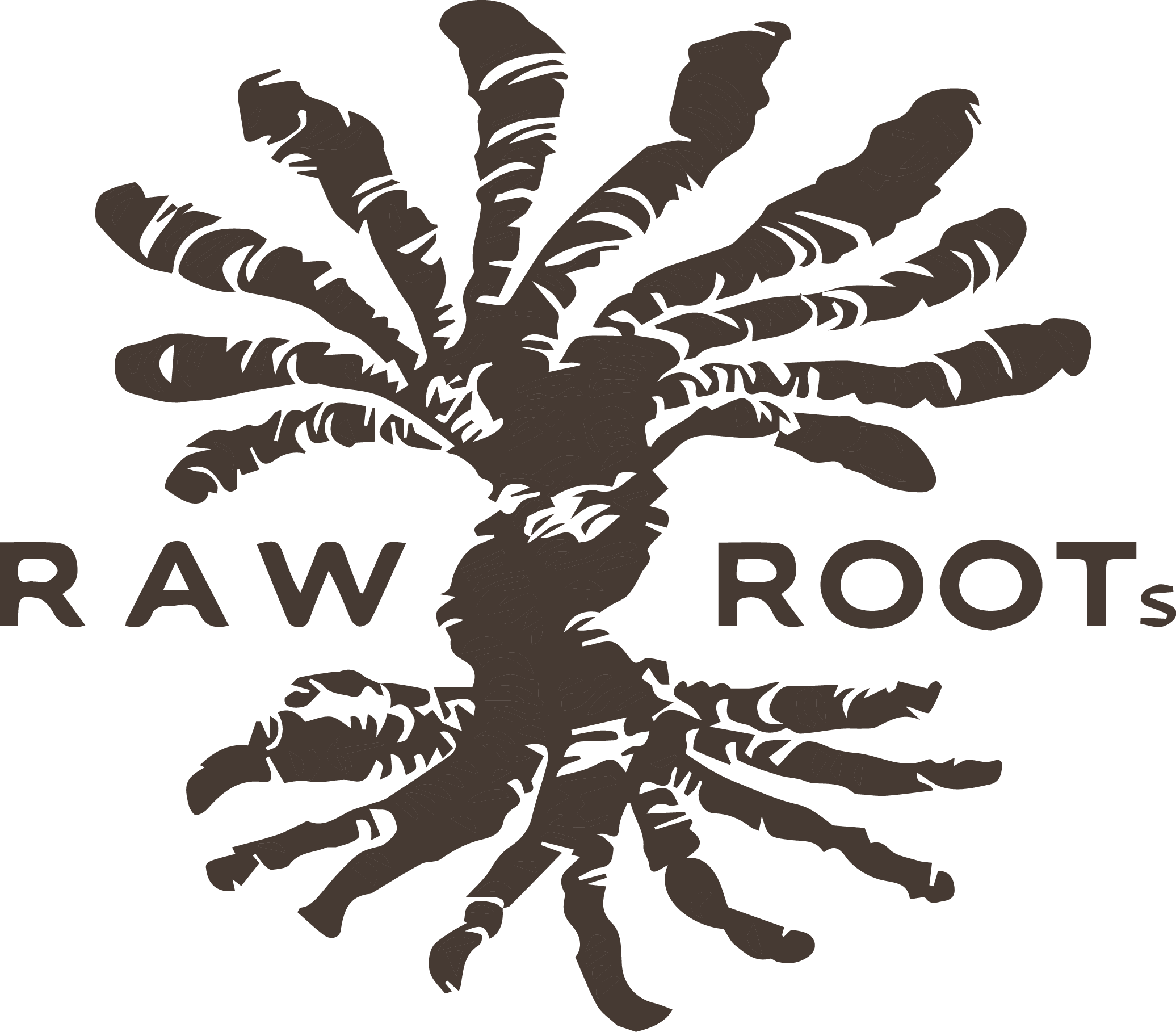The image features a detailed design, likely a logo for a company named "Raw Roots." The artwork, rendered in dark brown, is set against a white background and resembles a stylized tree. This abstract tree is split into two main sections: the top part, which fans out into ten tendrils that could be seen as branches or dreadlocks, and the bottom part, which mirrors this structure with root-like extensions. The tendrils are jagged and textured with white lines that accentuate their form. The central portion acts as a curved tree trunk connecting the two halves. On either side of this central trunk, the words "RAW" and "ROOTS" are displayed in uppercase black text, with the 'S' in "ROOTS" notably smaller. This intricate and symmetrical design creates an intriguing fusion of natural and human-like elements, exemplifying the concept of raw roots both visually and textually.